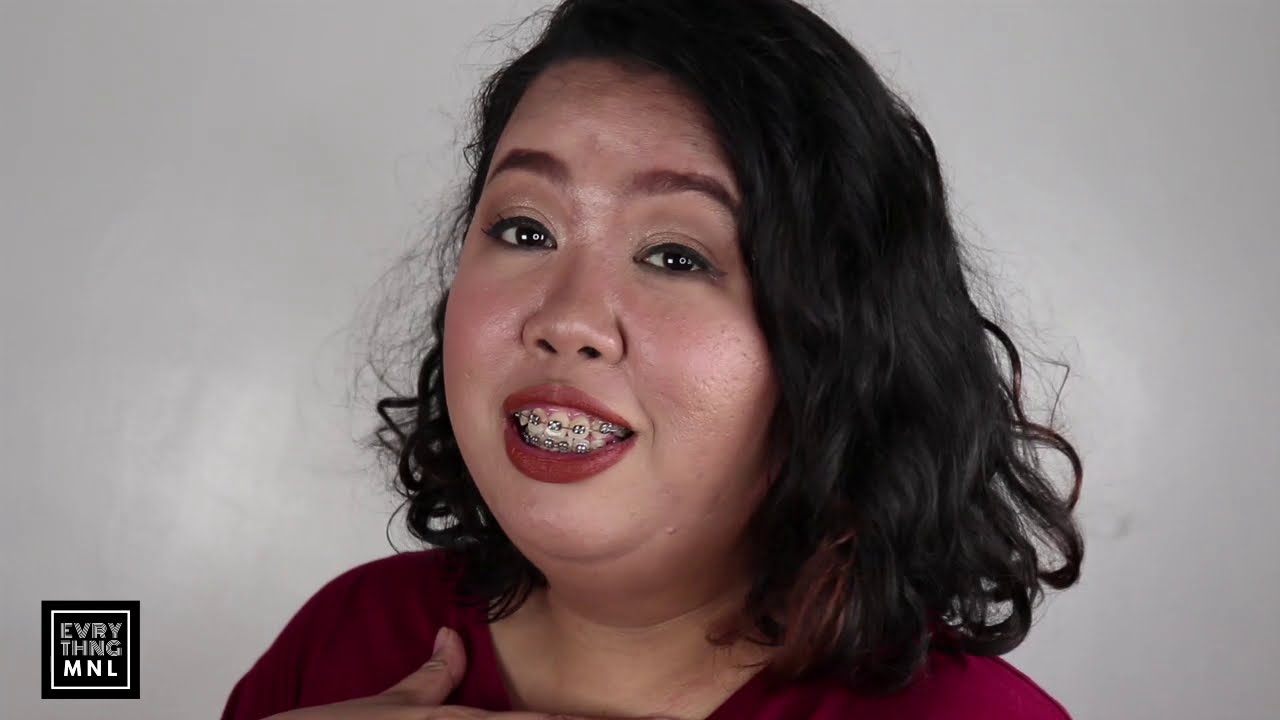This image is a close-up photograph of an Asian woman, from about the shoulders up, set against a light gray background with subtle highlights. The overall composition is a horizontal rectangle, roughly twice as wide as it is tall. The woman, who has a slightly overweight build, faces the camera with her head subtly turned to the left, offering a direct yet gentle gaze. Her shoulder-length hair is predominantly black with hints of lighter brown, indicative of dye, and has a slight wave, possibly styled. She wears a deep red or maroon shirt and red lipstick, complementing her appearance. Her mouth is open in a smile, revealing shiny silver braces on both her upper and lower teeth. In the bottom left corner of the image, within a black square outlined in white, are the words "EVRY THNG MNL" in gray and white lettering, suggesting some form of logo or branding.